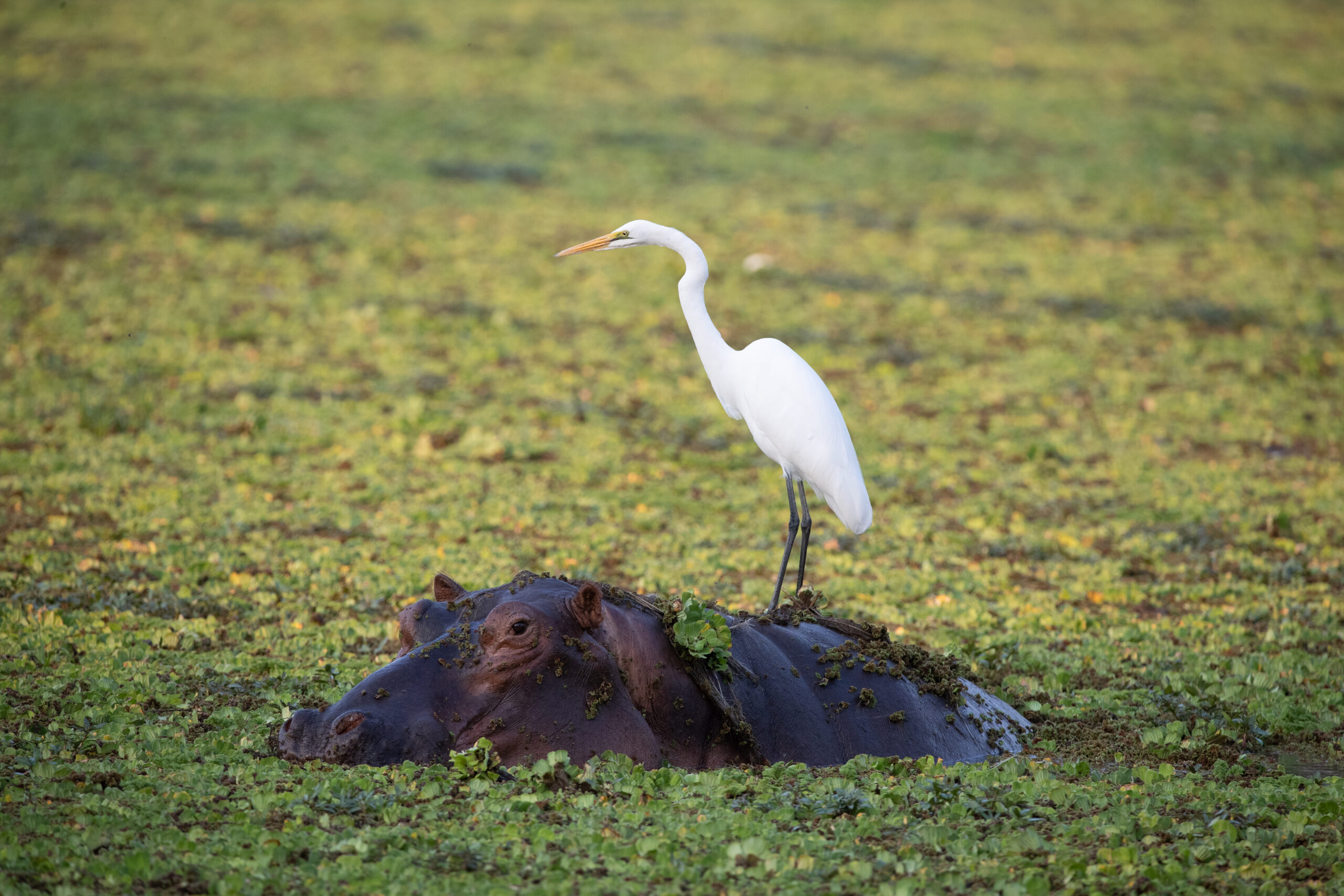In this detailed scene, a white bird, possibly a heron or crane with a long, yellow-orange bill and long, black legs, stands regally on the back of a hippo. The hippo, mostly submerged in what appears to be a shallow, plant-covered body of water, has its large, dark body and head visible above the surface, with distinct pinkish areas around its nostrils, eyes, and ears. The surrounding water is so densely covered with green vegetation that it almost resembles a grassy surface. The bird's slender, curved neck and prominent beak face to the left, and its small dark eyes are intently observing its surroundings. As the hippo moves through the water, creating a trailing path, the scene is captured with a shallow depth of field, rendering the background a soft, blurry green, emphasizing the subjects in the foreground.